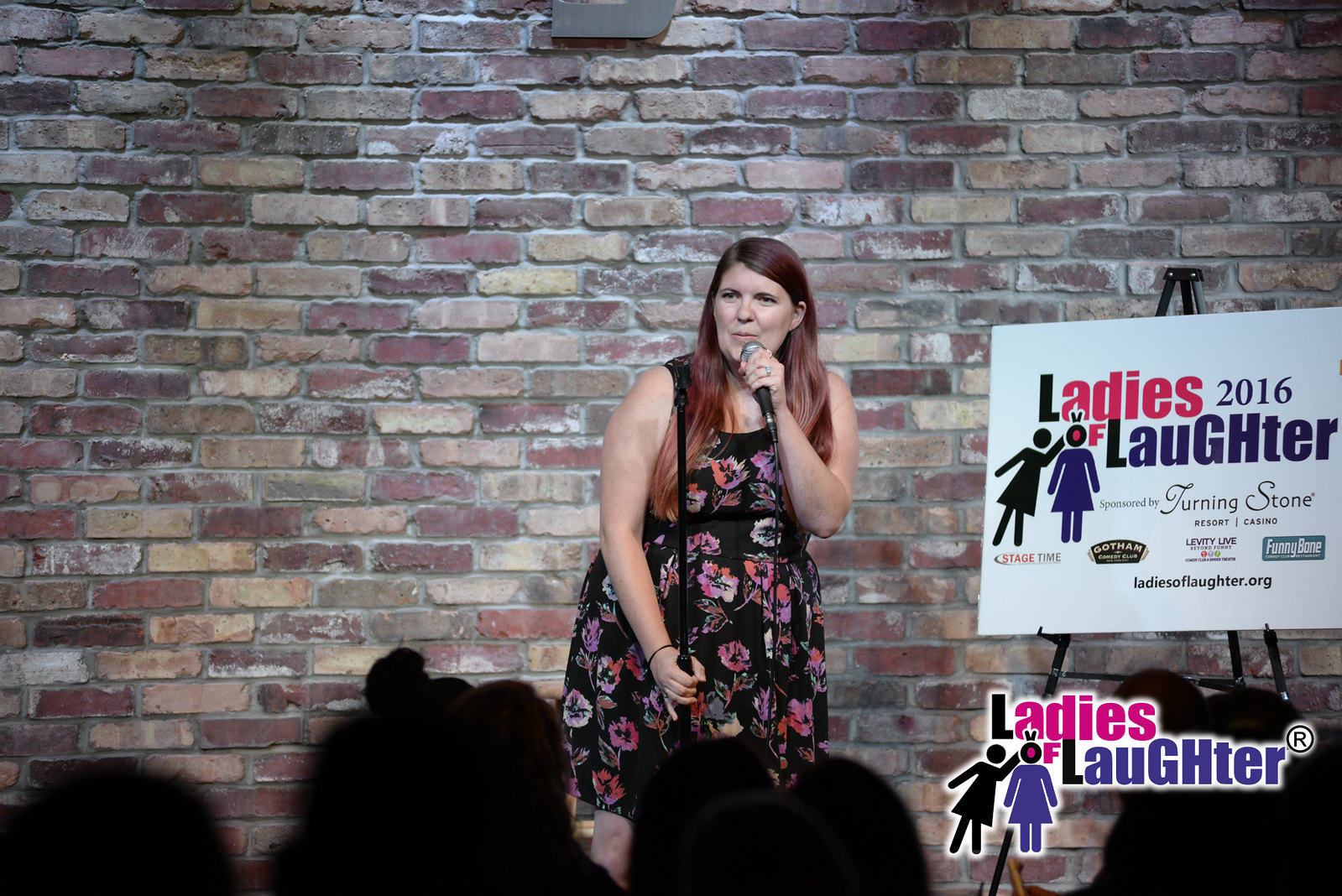In this photograph taken at a comedy event, a white woman in her 30s, possibly a stand-up comedian, stands at the center of the image. She has dark red dyed hair, styled into loose waves, and wears a black dress adorned with a colorful floral pattern featuring red, purple, and white flowers. She is slightly crouched, looking off to the left while holding a microphone with one hand and grasping the black microphone stand with the other. The backdrop is an old-school brick wall with a mix of reddish-brown and light brown bricks highlighted by gray cement.

To the right of the performer, there's a black easel displaying a white sign that reads "Ladies of Laughter 2016." The sign features a unique logo where the "O" in "OF" forms the head of a purple stick figure in a dress, reaching out to another black stick figure on the left. Below the main title, the event is noted to be sponsored by Turning Stone Resort Casino, with additional small logos of other sponsors such as Stage Time, Gotham Comedy Club, Levity Live, and Funny Bone. The event's website, ladiesoflaughter.org, is also listed. At the bottom of the image, silhouetted heads of the audience members can be seen, indicating their attention toward the comedian on stage. The logo for Ladies of Laughter, depicted with black and purple stick figures and colorful lettering, is also present at the bottom right of the photograph.